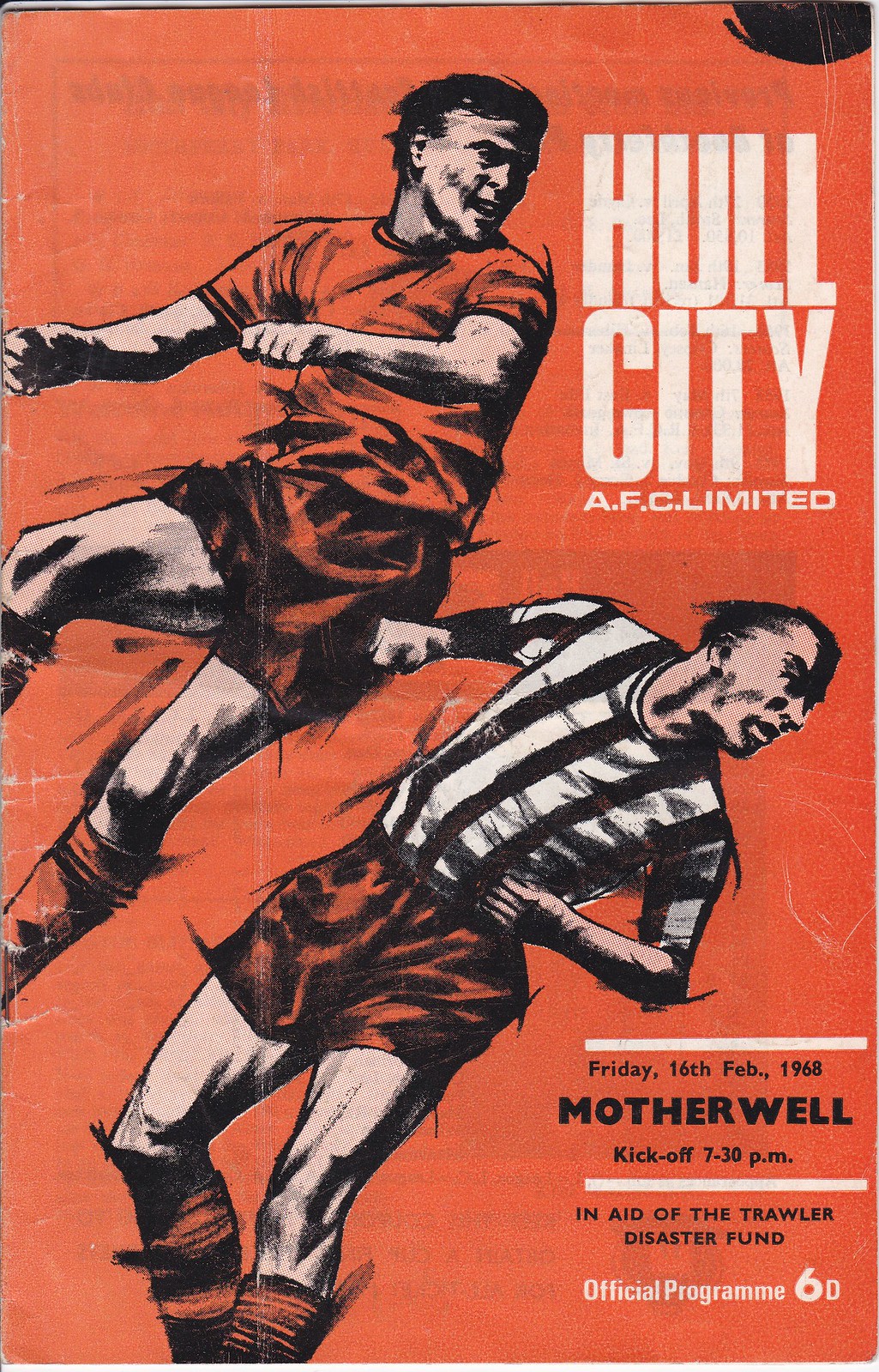The image is the cover of an old official soccer program, set against a red background. It prominently features an artistic depiction of two players in diagonal motion, seemingly heading toward a ball that's only partially visible in the upper right corner. One player, positioned higher, is dressed in a red jersey and shorts, with short brown hair, while the other wears a black and white striped shirt paired with red shorts. Both are looking to the left. In the upper right corner, large white block letters spell out "HALL CITY," with "A.F.C. Ltd." beneath in smaller white letters. The lower right corner contains a white horizontal bar with the text: "Friday, 16th February 1968, Motherwell, kickoff 7.30 p.m." Below it, another white bar reads, "In Aid of the Trawler Disaster Fund." At the bottom, in white letters, it says, "Official Program 6D."